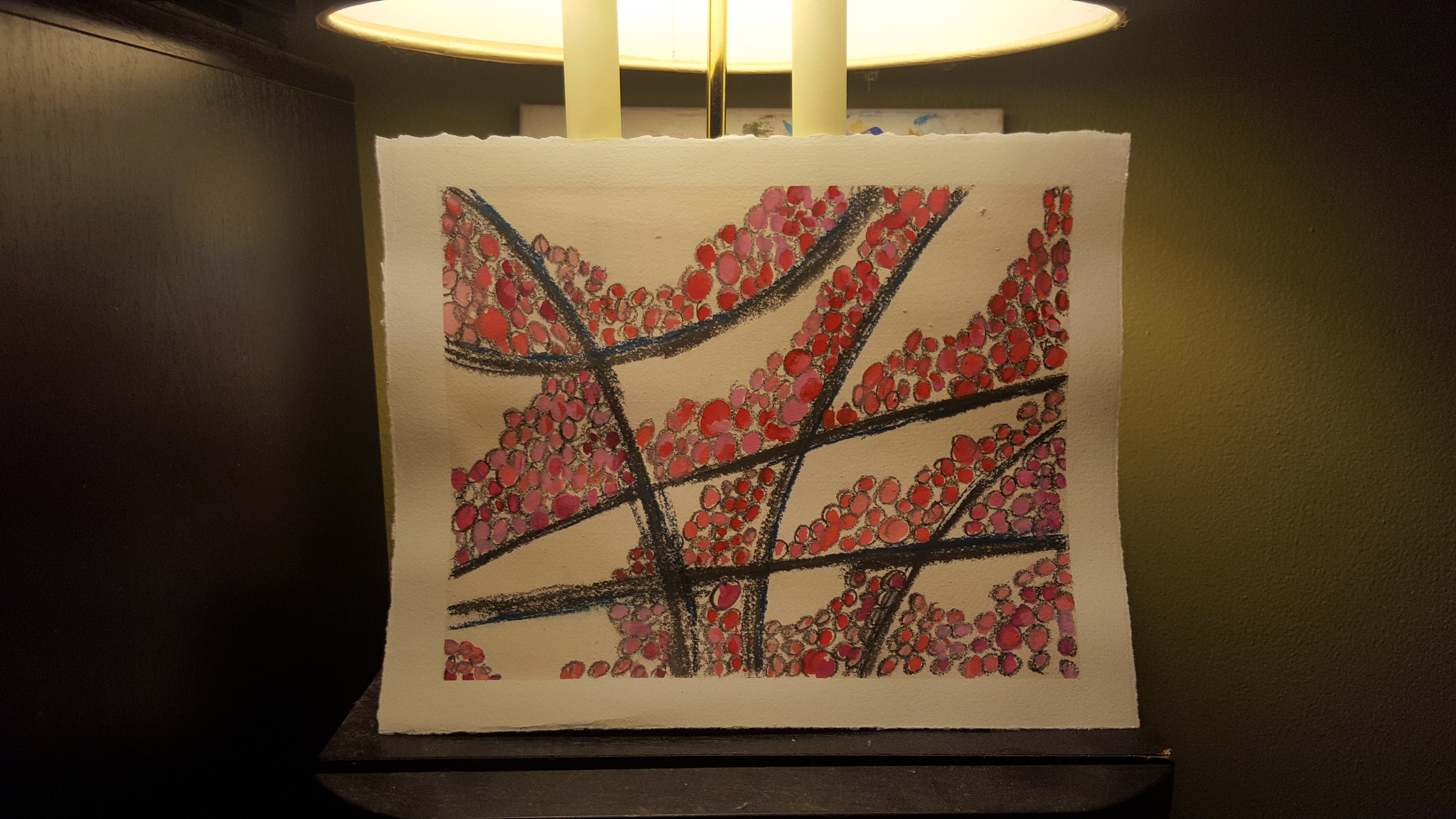An intricately sketched artwork, created with bold black colored pencils on a jagged-edged piece of white paper, rests propped against a lamp on an end table. The paper's uneven edges form a natural white border around the image. The sketch features an intricate web of criss-crossing black lines with various small, pebble-like circles nestled within the intersections. These pebbles, irregular in shape, are meticulously colored in shades of red and pink, adding a vibrant contrast to the monochromatic lines. The lamp, illuminated, casts a gentle light over the artwork, enhancing its colors and textures. The backdrop is a pale green wall, complementing the scene with a soft hue.